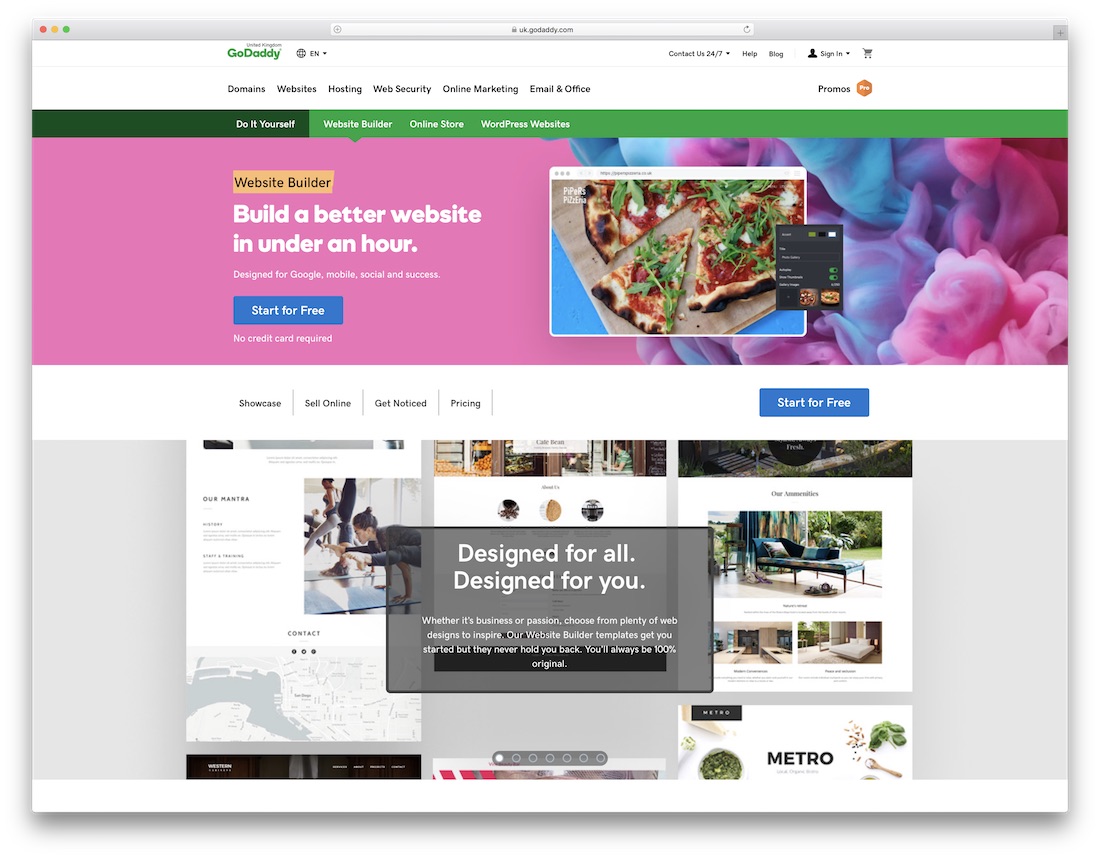**Caption:**

At the top of the image is a gray bar featuring the text "www.example.com" accompanied by three colored circles: red, yellow, and green, resembling traffic lights. The branding "GoDaddy" and options including "Contact Us," "24/7 Help," a lock icon, and "Sign In" are prominently displayed. Below this, Trevor Car is shown managing different aspects of web services like website hosting, web security, and digital marketing from his office.

A variety of website builder options are showcased, including a "Do-It-Yourself Website Builder," an "Online Store," and "WordPress Website." Several design elements such as rectangles are used to emphasize "Build a Better Website", "Designed for Google Mobile", and "Social Services," highlighting the platform’s user-friendly features. A promotional note indicates "No Credit Card Required" for trying the services.

The focal point shifts to a section advertising a sample website, "My First Pizzeria", complete with vibrant images of pizza and colorful flowers, emphasizing the aesthetics possible with the site builder. An inviting "Showcase Online, Get Noticed" message encourages users to explore. A blue rectangle with the text "Start for Free" offers an easy entry point into website creation. 

An inspirational section titled "Our Mantra" outlines the history, staff bios, and contact details, maintaining an approachable and helpful tone. Below, a white circle with different colored dots signifies user diversity and multiple design inspirations. The platform emphasizes designs fitting both business and personal passions, with tips and an arrow suggesting to "Get Started."

The image edges feature subtle shadow effects, contributing to a modern, sleek presentation perfect for creative inspiration and practical use.